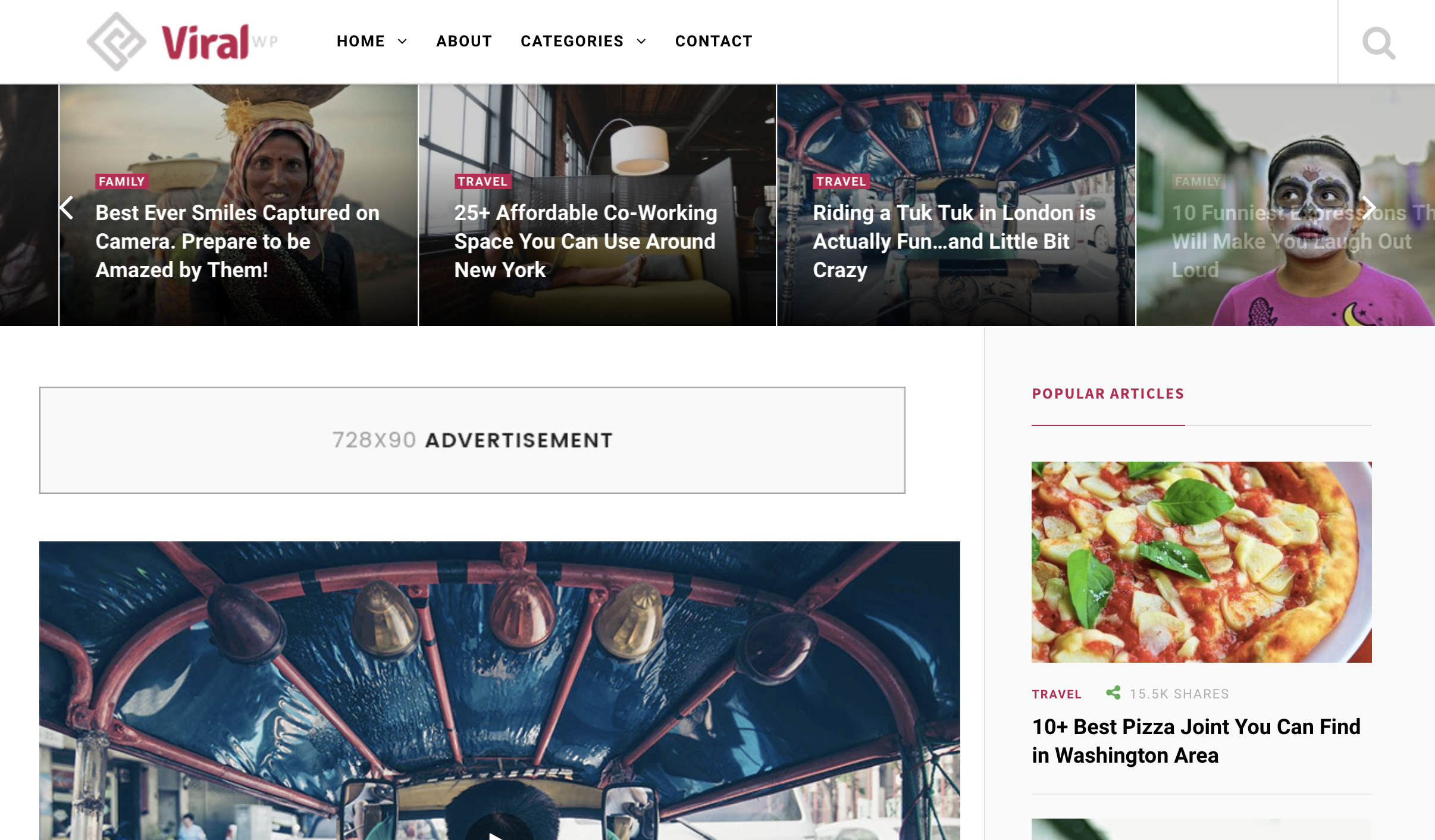The website depicted in the image is a vibrant and user-friendly tourism-oriented platform. Dominating the uppermost section of the page is a navigation menu featuring tabs such as Home, About, Categories, and Contact. The Home and Categories tabs are further enhanced with drop-down options, whereas the About and Contact tabs are standalone. Adjacent to the navigation on the top right is a search icon, facilitating easy content location for users. On the top left, the brand's visually prominent logo catches the eye, accompanied by the site name "Viral WP." The word 'Viral' is presented in bold red text with an uppercase 'V' followed by lowercase letters, while 'WP' appears in smaller uppercase letters positioned to the immediate right.

Below the site header, a carousel showcases four clickable articles, each accompanied by relevant tags. Two articles are tagged under 'travel,' while one is under 'family.' The family-tagged article, positioned on the left, is titled "Best Ever Smiles Captured on Camera. Prepare to be Amazed by Them." Adjacent to it, the first travel article is called "25+ Affordable Co-Working Spaces You Can Use Around New York." The second travel article, found at the rightmost position, intriguingly titles "Riding a Tuk-Tuk in London Is Actually Fun... and a Little Bit Crazy," inviting readers with a touch of suspense and adventure. The carousel arrangement ensures easy access to engaging and diverse content for visitors looking to explore various travel and lifestyle insights.